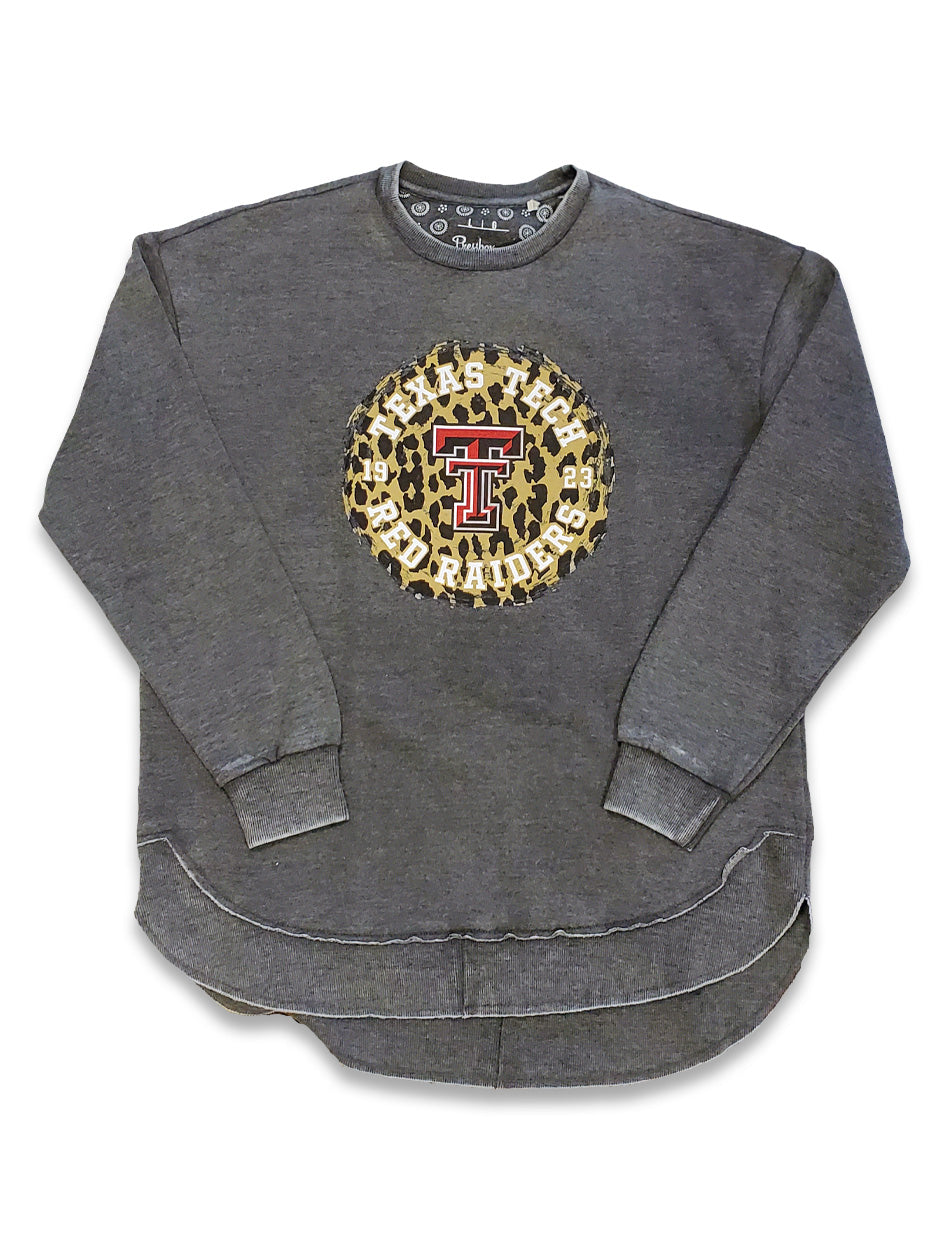This image depicts a dark gray women's sweatshirt, laid flat on a white surface, with the sleeves folded towards the middle. The sweatshirt prominently features a Texas Tech University logo at its center. The logo includes two red, three-dimensional Ts with a white outline, the larger T underneath the smaller one. Encircling the Ts is a leopard print design in black and yellowish-orange, along with white text that reads "Texas Tech" at the top and "Red Raiders" at the bottom. Additionally, the numbers "19" and "23" are positioned to the left and right of the Ts, respectively. The sweatshirt is a classic crew-neck style with a wide, thick hem at the bottom and elastic cuffs on the sleeves, providing a snug fit. The inside collar has small white designs, which appear to be circular but are too small to discern clearly.